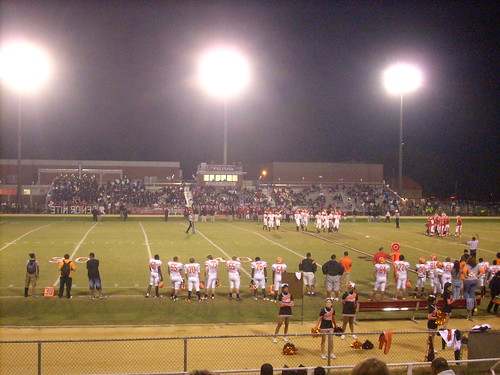This image captures a high school football game taking place at night under three bright stadium lights that illuminate the green grass field marked with white lines. The photograph is taken from the stands, showing a modest crowd of fans seated on bleachers and standing around the field. Two teams are present on the field: one team wearing white uniforms with red letters or numbers, and the other team also in white but with orange helmets, with some players holding their helmets. The players appear to be on a break, gathered in groups along with coaches and referees. Cheerleaders in black and red uniforms with matching pom-poms are positioned near a metal fence that separates the field from the spectators. Behind the well-lit field, a few buildings can be seen against the dark night sky. The image is bright and clear, enhanced by the stadium lights and the vivid colors of the scene.